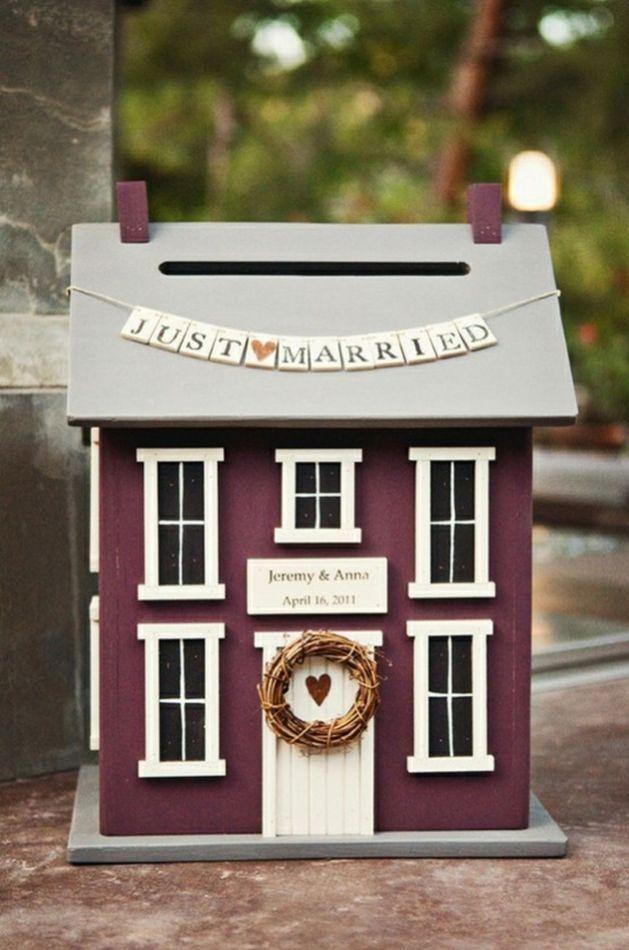The image depicts a detailed, custom-made miniature house, meticulously crafted to resemble a real home. The house itself is predominantly burgundy or maroon, featuring white windows and doors, with a gray roof and two matching maroon chimneys. A prominent feature of this quaint model is the wreath on the front door, which has a cut-out heart in its center. Above the door, an inscription reads "Jeremy and Anna, April 16, 2011," suggesting a significant date, likely a wedding. Adding to the celebratory theme, the roof has a message spelled out in what appear to be Scrabble tiles, reading "Just Married." There is also a slit in the roof, indicating that the miniature house might serve as a decorative card box for wedding greetings or monetary gifts. This intricately designed model portrays a heartfelt and personal touch, symbolizing the couple's cherished moments.